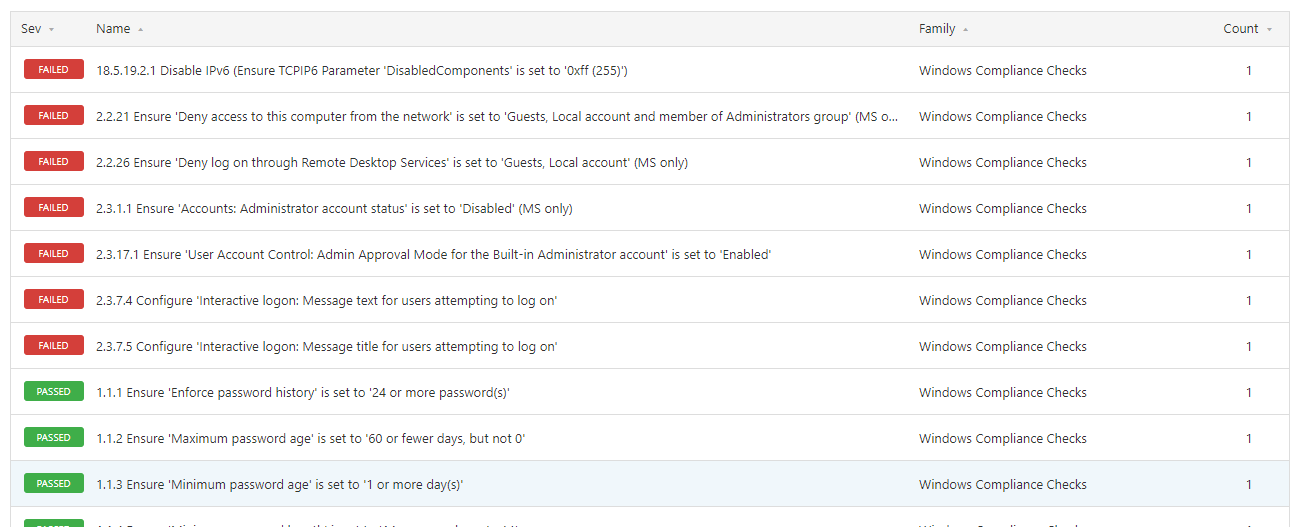The image depicts a minimalistic website layout featuring a gray navigation bar at the top. On the left-hand side of this bar, the acronym "SSEV" is prominently displayed. The navigation bar also contains three sections labeled "Name," "Family," and "Count."

Beneath the navigation bar, the rest of the page consists of a list format. Each item on the list includes colored status bars, where red indicates a "failed" status and green signifies a "passed" status.

For example, under the "Name" column, the entries include various compliance checks such as "Ensure accounts administrator," "Account status is set to disabled," and others. Adjacent to these entries, the "Family" column consistently displays "Windows compliance checks," emphasizing the system’s focus on Windows-based evaluations. In the "Count" column, each entry is marked with the number "1."

Most of the entries are presented on a white background, with red or green status bars signifying their current compliance status. A notable exception is one entry at the bottom of the list, which has a distinct light blue background and a green "passed" status bar. This particular entry details the compliance requirement "Ensure minimum password age is set to one or more days."

Overall, the image conveys a straightforward and structured compliance checking interface, with clear indicators of system status and specific compliance criteria.